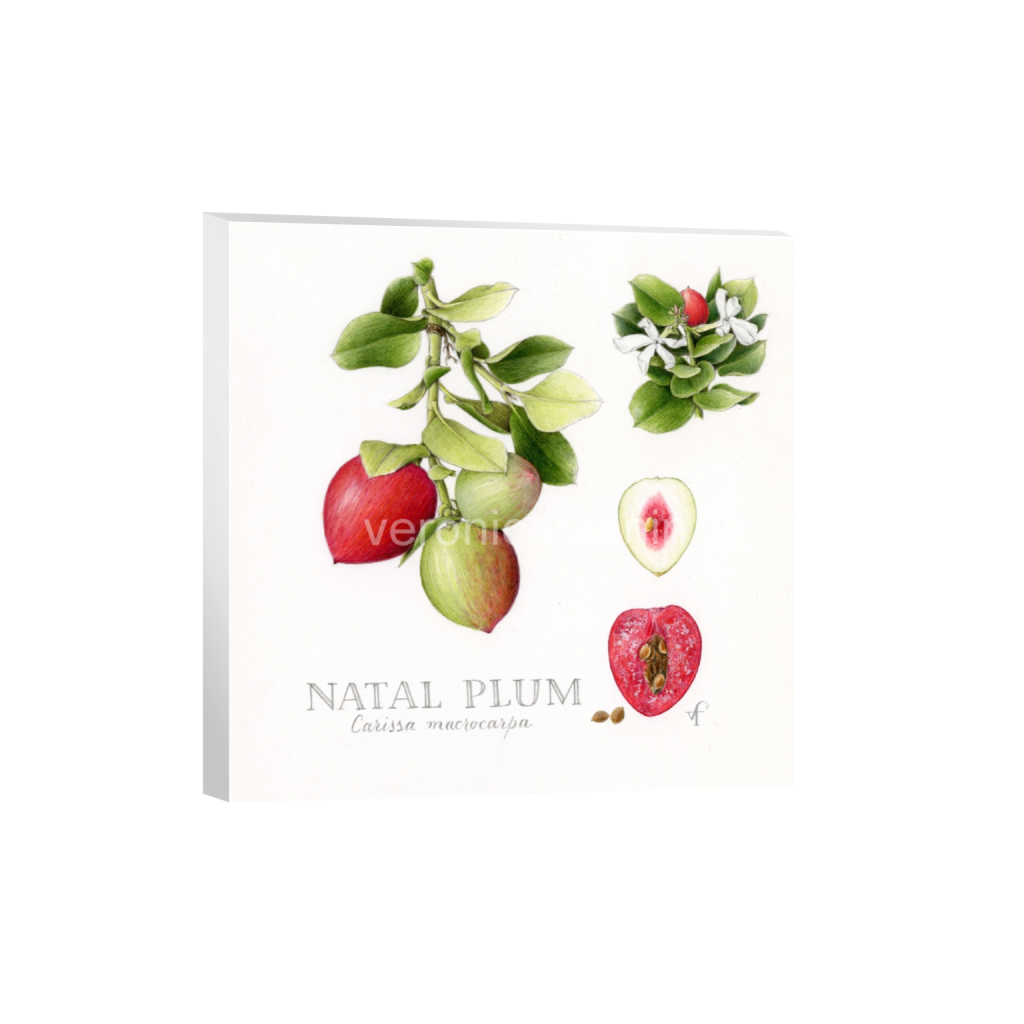The image portrays a detailed, colorful illustration against a white background, without any border. In the bottom left-hand corner of the image, the text "NATAL PLUM" is displayed in all caps in gray, with the scientific name "Carissa macrocarpa" beneath it in smaller print. This image comprehensively showcases different views of the natal plum and its plant.

In the upper left section, a green stem with light and dark green leaves extends downward, adorned with three fruits: one red, resembling a red onion, and two green-tinged fruits with touches of red. 

The upper right corner features a cluster of green leaves with white flowers, accompanied by a small, round red bulb. 

On the middle right side, a top view of a sliced fruit reveals a pink center filled with tan seeds. 

Finally, in the lower right corner, there's another slice displayed, characterized by a dark pink to almost red exterior with brown seeds in the middle. 

Overall, the image is bright, clear, and rich in details, with distinct visual representation of both ripened and raw natal plums and various parts of the plant.